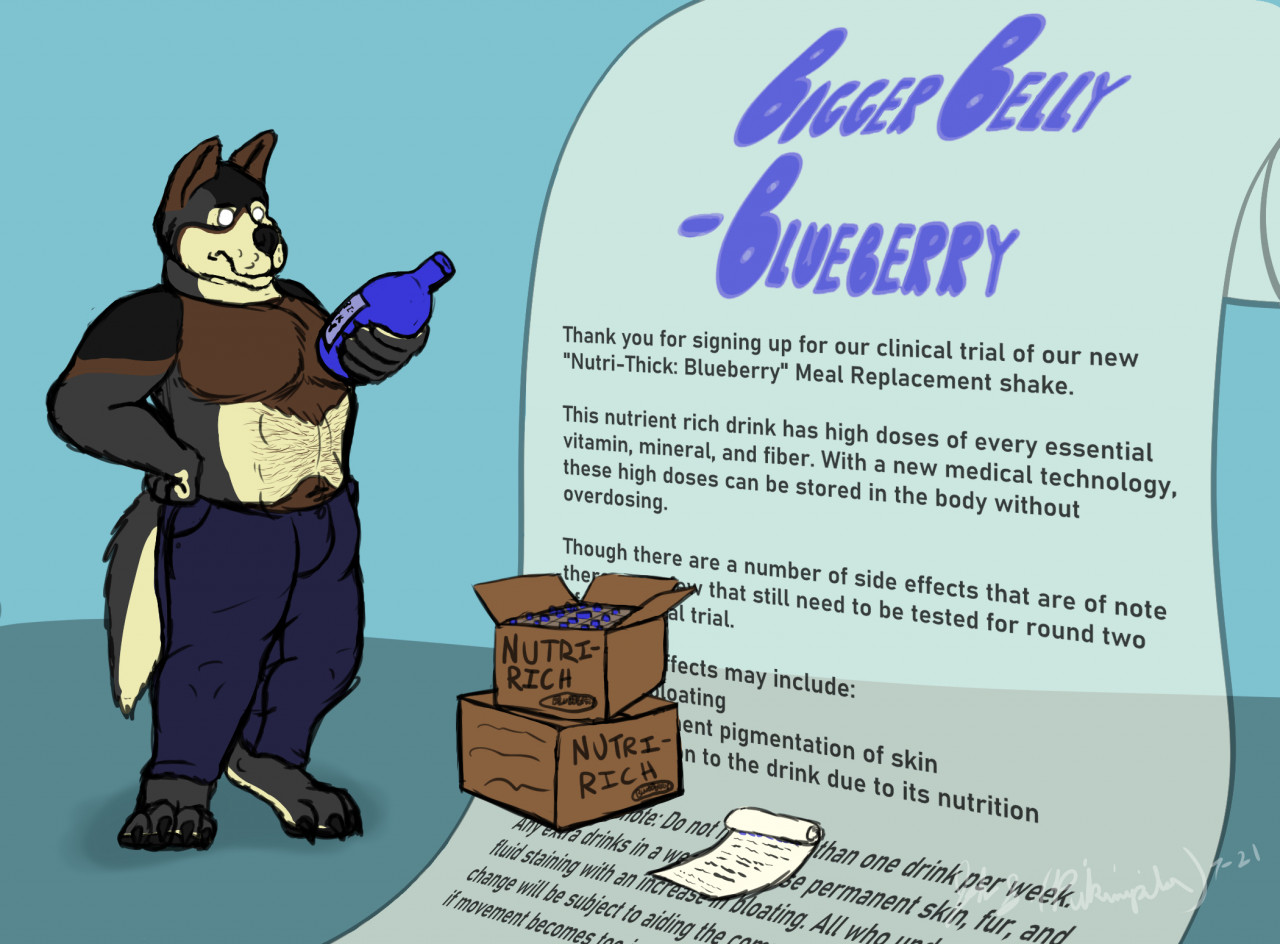The image depicts a cartoonish, anthropomorphic animal standing on its hind legs. The character, which appears to be a muscular fox or bear-like creature with pointed ears and a big bushy tail, has distinct human features including white abs exposed among its brown fur and gray feet. The character's brown ears and gray hands are visible as it holds a blue bottle. The figure is wearing blue jeans but no shirt, exposing its toned chest, which is a lighter color relative to its fur. The character is fixated on the bottle. 

To the right of the character, an unrolled, scroll-like page in a light blue hue displays a promotional text. At the top, it reads in blue font, "Bigger Belly Blueberry." The subsequent text in black font begins with, "Thank you for signing up for our clinical trial of our new Nutri-Thick Blueberry meal replacement shake." The text goes on to explain the nutrient-rich drink, emphasizing its high doses of essential vitamins, minerals, and fiber, and mentioning a new medical technology that allows these nutrients to be stored in the body without causing overdose. However, it also notes some side effects. The scroll's complete message is partially obscured by two boxes labeled "Nutri-Rich," featuring the same blue liquid bottles depicted in the character's hand. Another smaller white scroll with black writing overlaps the larger scroll.

The overall theme and aesthetic of the image are promotional, centered on the Nutri-Rich product, with vibrant and engaging visuals designed to captivate viewers.